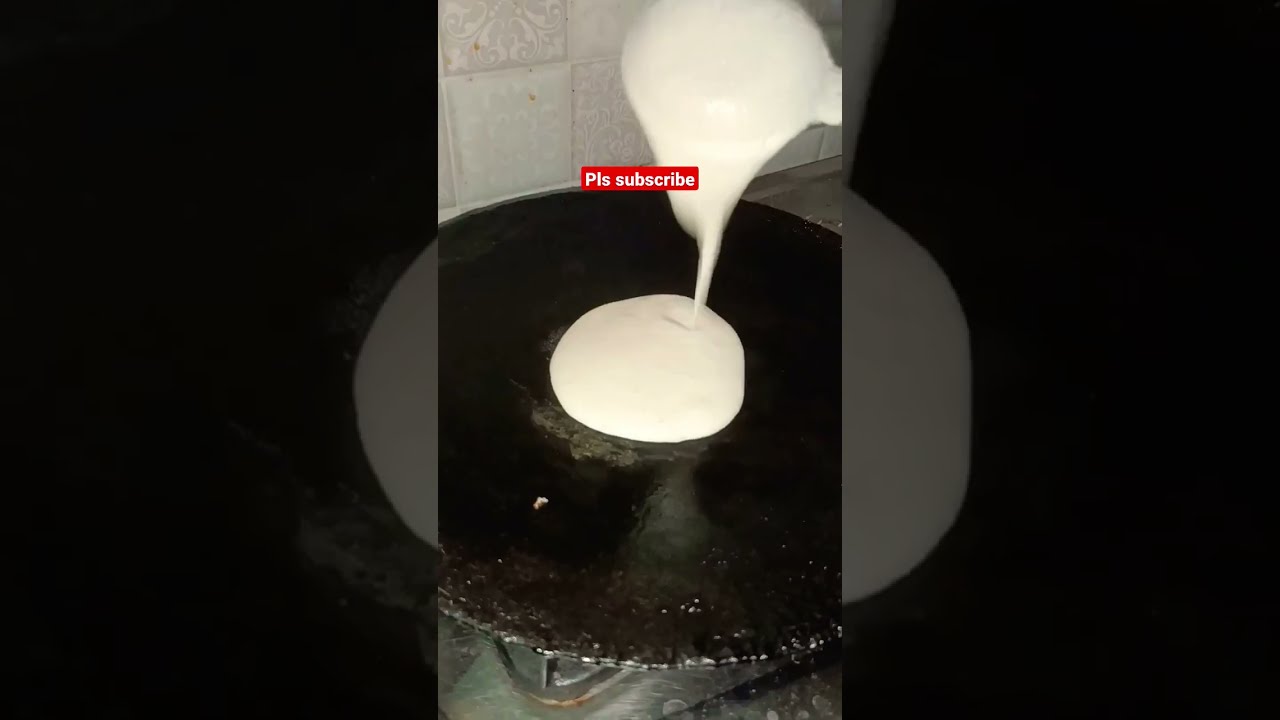This image captures a close-up scene in a kitchen, focusing on a round, flat pan, likely on a stove burner visible at the bottom. In the center of the shot, a large spoon is dripping pancake batter, creating a circular pattern as it falls onto the pan, suggesting the preparation of a pancake or possibly a large single pancake. The backdrop of the image features white tiles, hinting at a kitchen setting. Superimposed on the top central part of the image is a red bar with white text that reads "PLS subscribe," indicating a promotional element, possibly for a cooking channel. The image composition includes an artistic touch, as the edges on the left and right sides display an enlarged, darkened version of the batter and pan, adding a unique texture to the overall presentation.